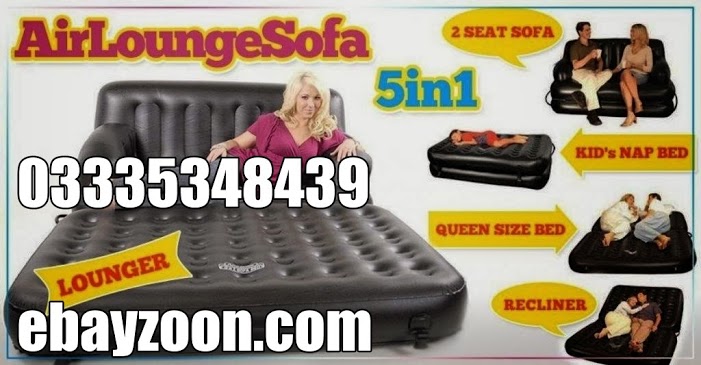This image is an advertisement for a versatile inflatable lounge sofa, branded as the Air Lounge Sofa, available on EbayZoon.com and featuring a prominent contact number, 0333-534-8439. The ad showcases the sofa's five-in-one functionality, demonstrating it in various configurations including a two-seat sofa, a kids' nap bed, a queen-size bed, a recliner, and a lounger. The main visual on the left side of the ad features a black inflatable lounge sofa upon which a woman in a pink dress is lounging comfortably. Adjacent to this are smaller images illustrating each configuration: a couple enjoying coffee on the two-seat sofa, a child napping on the kids' nap bed, a pajama-clad couple on the queen-size bed, and another couple cuddling on the recliner. The ad emphasizes the sofa's multi-use design, making it adaptable for different lifestyle needs.